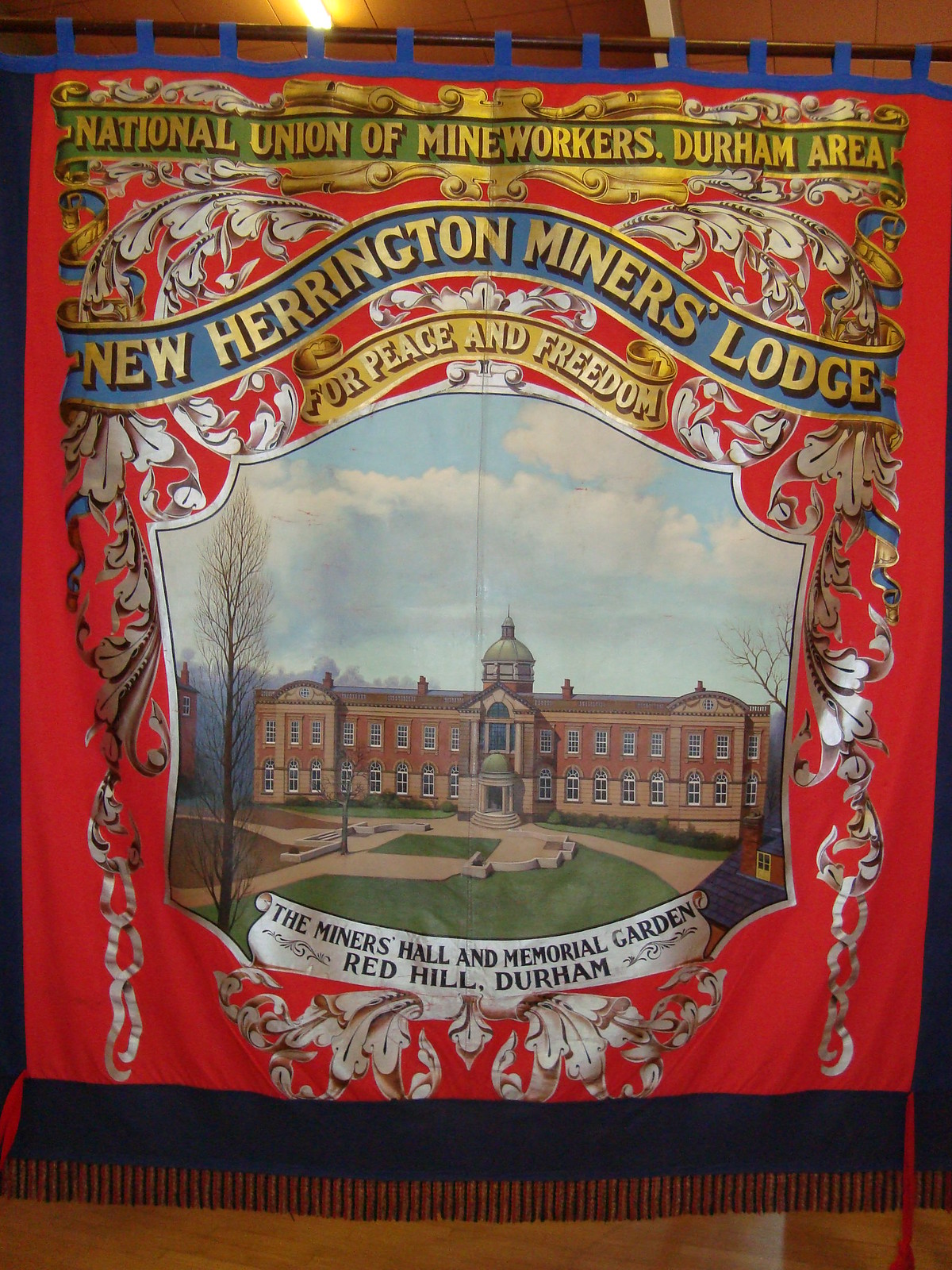The image is a detailed photograph of an indoor scene featuring a prominent red banner hanging from a black metal pole, supported by blue strips. The banner has a vibrant red background with intricate flowery designs around a shield. Across the top, in gold letters, it reads "National Union of Mine Workers, Durham Area." Below this, a wavy blue banner with gold print states "New Harrington Miners Lodge," followed by a smaller gold ribbon that reads "For Peace and Freedom."

The central shield on the banner depicts a blue sky with tall, leafless trees surrounding a two-story brick building. This building has an arched area in the center and a small spire on top, suggestive of a miners' hall or a college-like structure. Near the bottom of the shield, a white scroll-like banner with black print says "The Miners Hall and Memorial Garden, Red Hill, Durham." The lower edge of the banner is adorned with a blue border and a fringe of tightly packed black strings. The background scene includes brown wooden ceiling slats and a white light visible about a third of the way from the left.